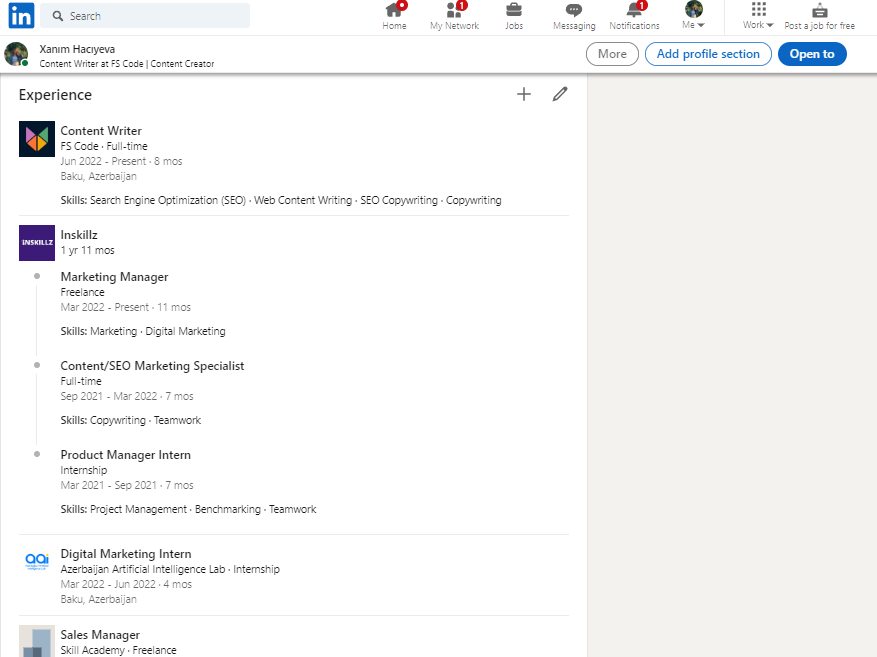This image is a detailed screenshot of an individual's LinkedIn profile page, showcasing their professional resume. At the forefront, it highlights their current role as a Content Writer, a position they have held since June 2022 and continue to occupy to date. Prior to this, they worked at InSkills in various capacities, including Marketing Manager, Product Manager Intern, and Content Marketing Specialist. Further down, their background includes internships as a Digital Marketing Intern, and a stint as a Sales Manager.

Captured from a computer screen, the visual layout includes the familiar LinkedIn interface features situated at the top right corner. These features consist of navigation buttons for Home, My Network, Jobs, Messaging, and Notifications, alongside the user's profile picture and a link to their profile. The screenshot effectively encapsulates the organized structure of their career journey as presented on the LinkedIn platform.